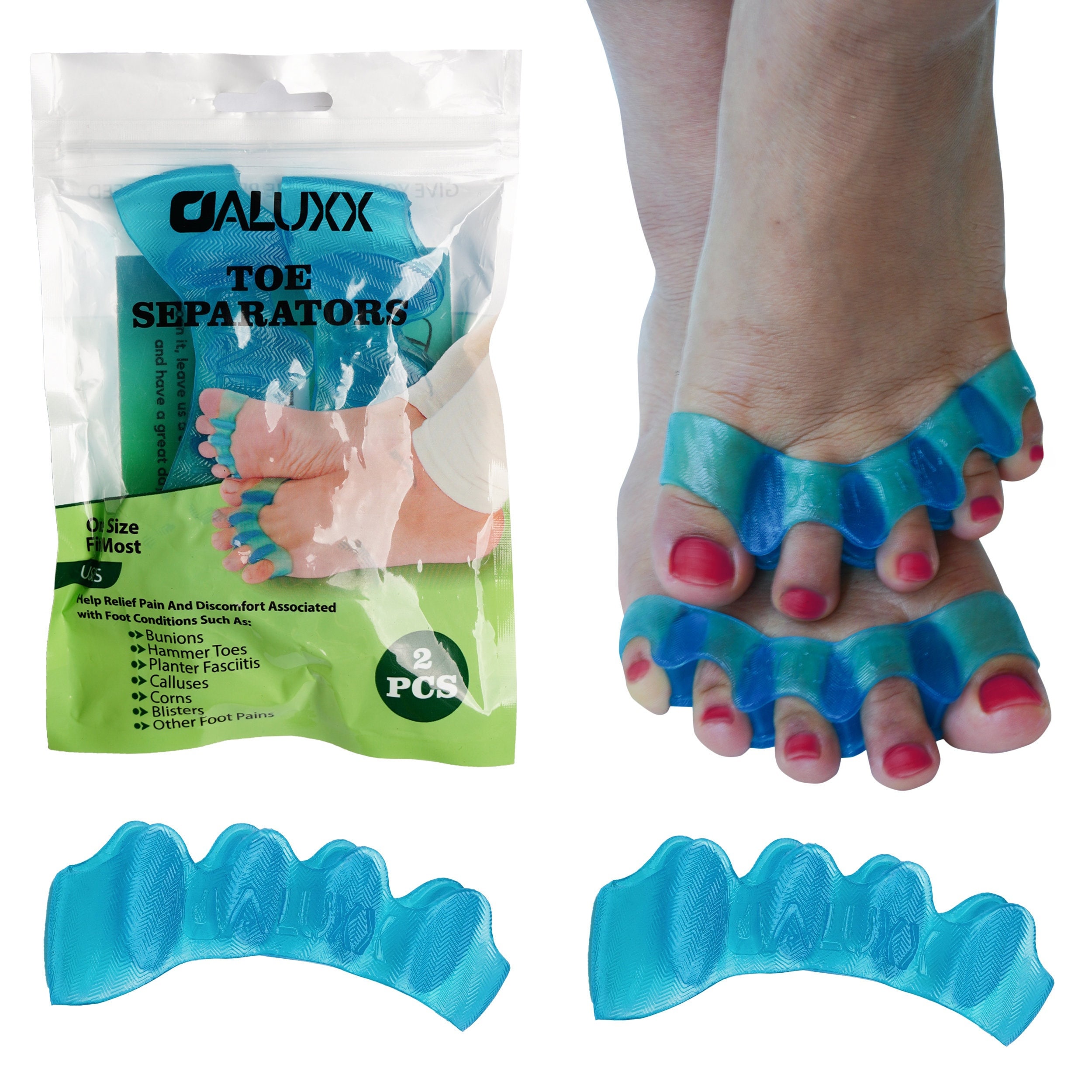The image depicts a light-skinned woman with polished red toenails using bright blue toe separators that are looped over each of her toes, effectively spreading them apart. One foot is flat on the ground while the other rests on top of it, showcasing the product in action. On the left side of the image, there is a clear and green package labeled "Aluxx Toe Separators," which contains two pieces and claims to relieve pain and discomfort associated with various foot conditions, including bunions, hammer toes, plantar fasciitis, calluses, corns, and blisters. The package also mentions that the product "fits most sizes." Below the feet, the image features two standalone blue toe separators, highlighting their material and functionality. The feet appear aged, adding context to the product's intended use for relief and comfort.